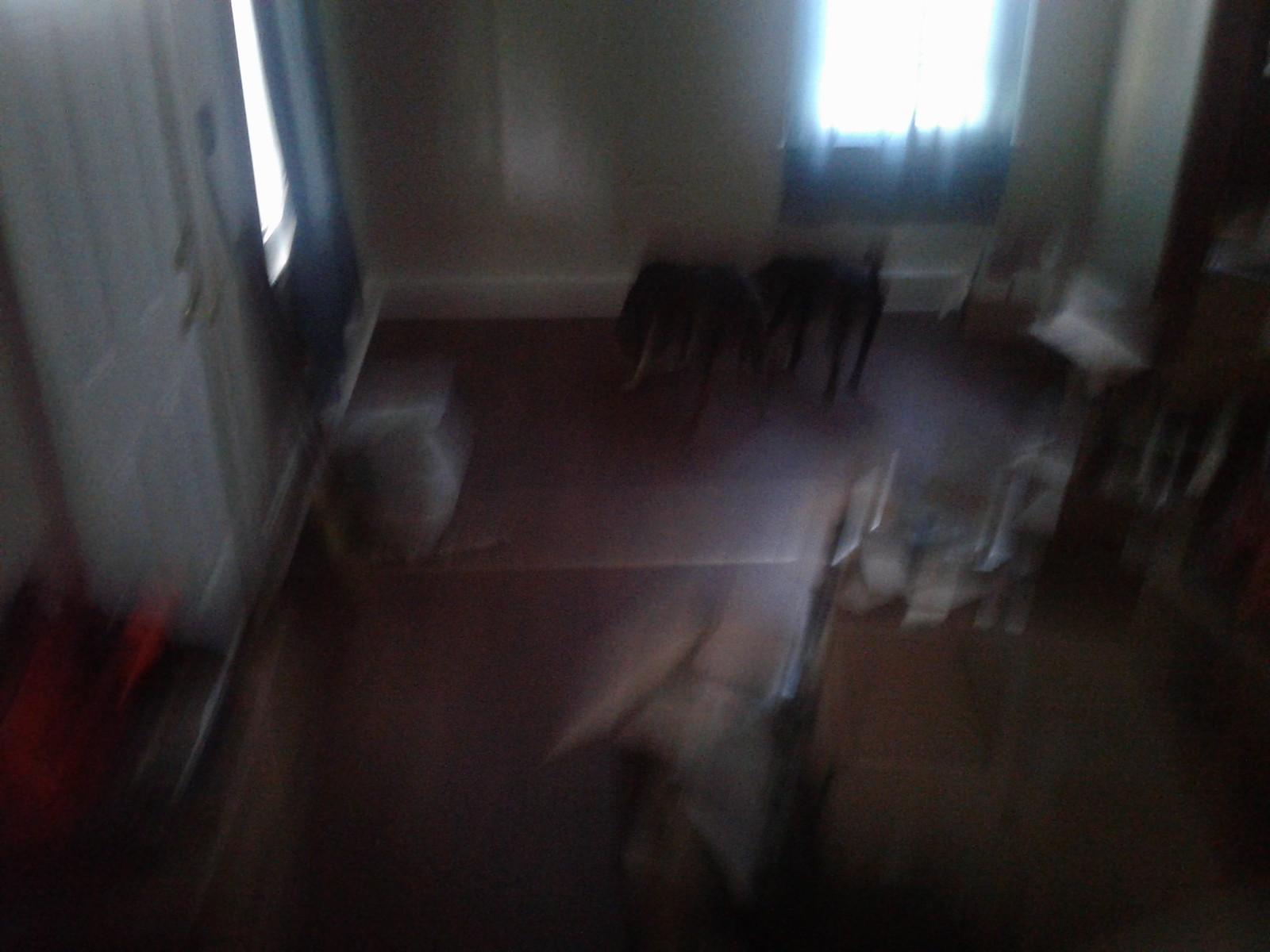The image is a blurry, low-quality photo of a room, likely taken from an elevated angle, possibly a staircase or the second floor, looking down onto a wooden floor. The flooring is brown, and scattered across it are two black dogs. The left wall of the room features a black container with something red on top, next to a white door with a bit of white wall visible beyond it. A window, partially covered by a blue curtain, appears on the back wall, through which some light is shining. A clear plastic bag, which looks like trash, is placed in front of the window. Below the window stands one of the black dogs, while the other is slightly to the left. Further along the back wall is a desk with some papers on it, positioned near the top right. The right side of the desk is cluttered, and nearby, there's another set of boxes, although it is difficult to distinguish contents due to the photo's blurriness.